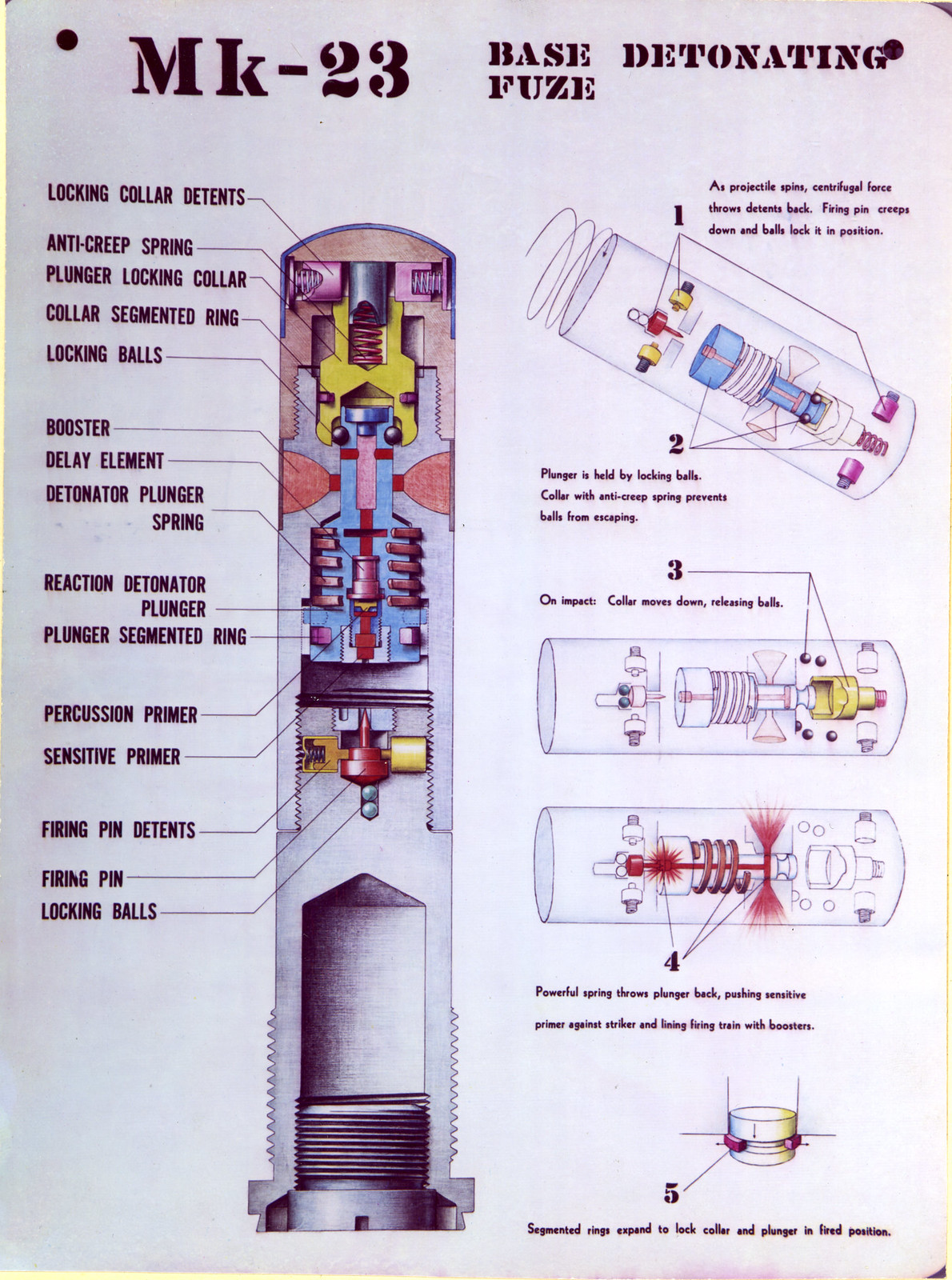The image depicts a detailed technical illustration that resembles an advertisement from a magazine or newspaper. At the top, it prominently features the text "MK23 Base Detonating Fuse." The central focus is a large, detailed illustration of the MK23 fuse, which is cylinder-shaped and silver, resembling a tube. Detailed annotations with lines and labels identify various components of the fuse, including the locking collar detents, anti-creep spring, plunger, segmented ring, locking balls, booster, delay element, detonator, and firing pin among others. To the right of this main diagram are four smaller, less colorful illustrations of the same object, labeled 1 through 5, showcasing different views or stages. Each part of these illustrations is also meticulously labeled with bullet points, indicating the inner workings of the fuse, from the percussion primer to the sensitive primer and beyond.